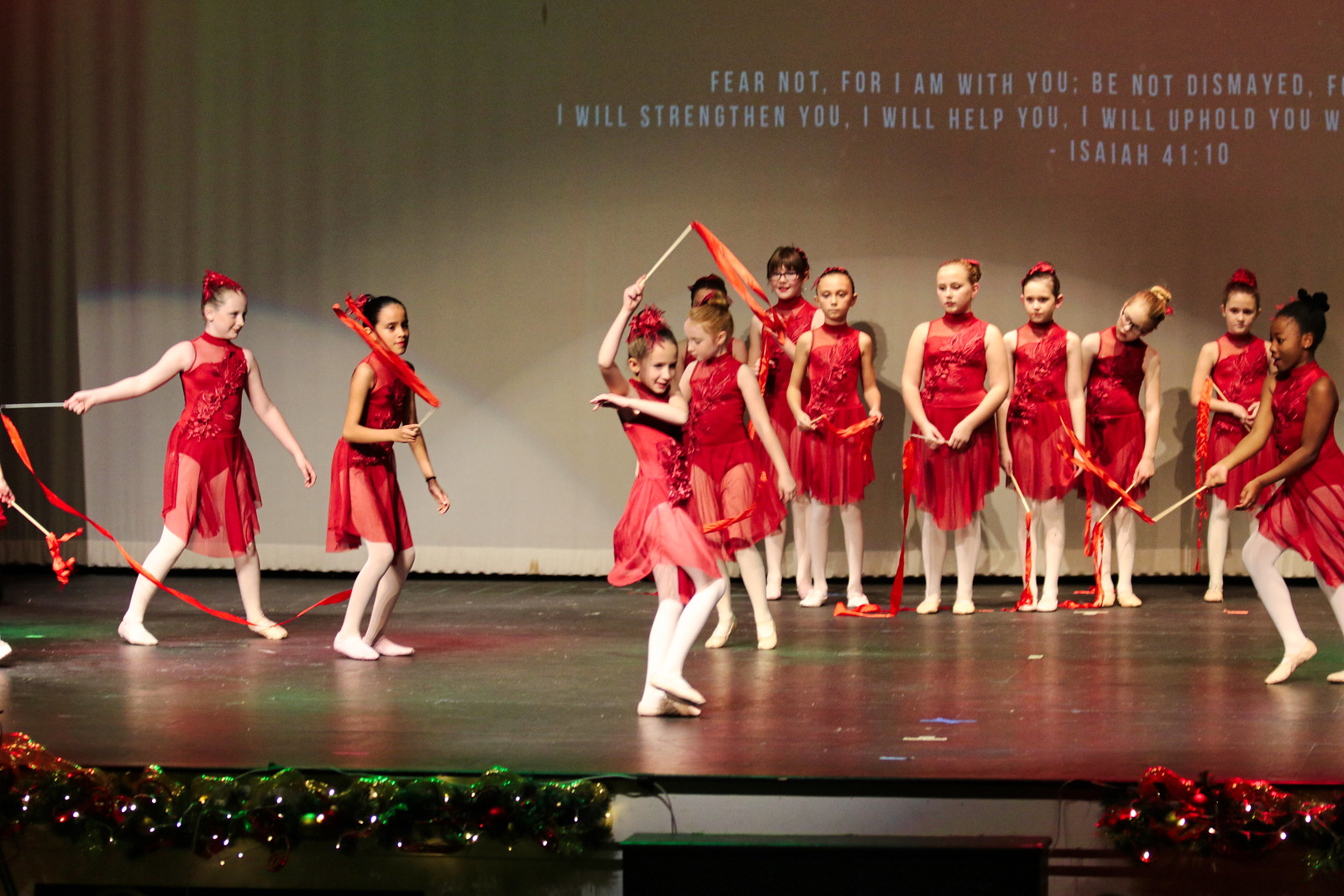In this indoor photograph, a group of 10 to 15 young girls, all seemingly under the age of ten, stand on a rectangular stage adorned with festive garland interwoven with Christmas lights along its front edge. Each girl is dressed in a vibrant red sleeveless leotard paired with a sheer red skirt and white tights. They complete their outfits with white shoes. The girls are performing a dance routine, brandishing sticks decorated with red or orange streamers.

At the center of the stage, one girl is actively waving her stick in the air, capturing the attention of her fellow performers who are mostly positioned towards the sides, watching intently. The stage features green steps just right of center and is set against a backdrop of a large light-colored curtain. Projected onto this curtain, in blue text, is the inspirational biblical verse: "Fear not, for I am with you; be not dismayed, for I will strengthen you, I will help you, I will uphold you, Isaiah 41:10." The composition of the group is diverse, including girls of varying ethnic backgrounds, predominantly Caucasian with at least one of African descent, all united in their spirited performance.